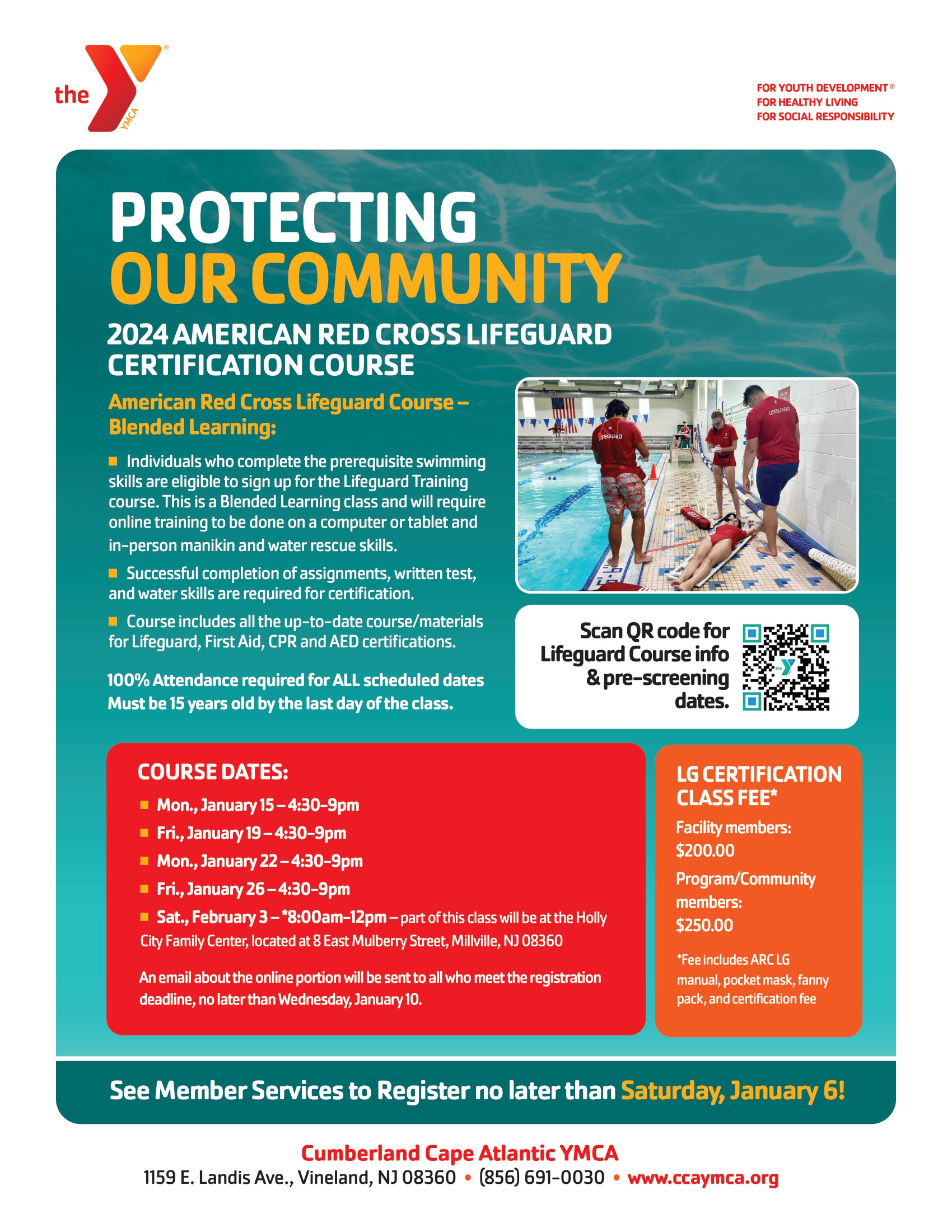The image is an advertisement for the Cumberland Cape Atlantic YMCA located in Vineland, New Jersey, promoting the 2024 American Red Cross lifeguard certification course. The top of the flyer displays "The Y" and the message "Protecting Our Community." The flyer justifies vibrant colors including aquamarine green, red, orange, and yellow. 

Central to the flyer is an image of three lifeguards wearing red shirts standing next to a pool, attending to a woman in a red swimsuit who is laid out on the floor beside the pool. The text details the lifeguard certification course, mentioning it is a blended learning program with 100% attendance required for all scheduled dates and that candidates must be at least 15 years old by the last day of the class.

The flyer includes multiple bullet points elaborating on the training, testing, and certification process for the course. There are two informational boxes colored red and orange, each containing details about the course dates and fees. A QR code is provided for additional course info and pre-screening dates. At the bottom of the flyer, it says to see member services to register no later than Saturday, January 6, followed by the YMCA's full name, address, phone number, and website.